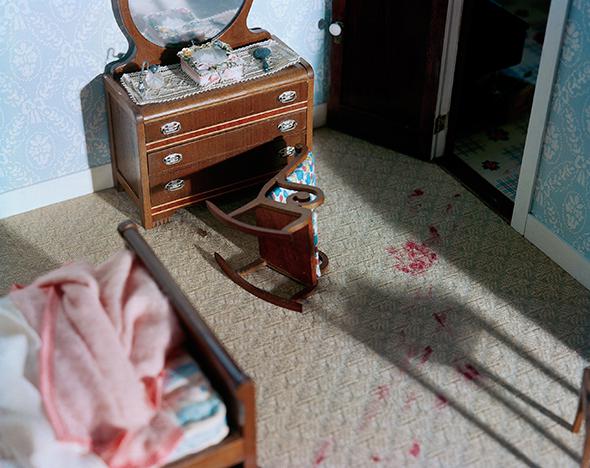The image depicts an intricately detailed scene resembling a crime scene, but with a scale model quality, suggesting it might be a staged dollhouse setting. The perspective is a wide vertical rectangle, looking down onto a bedroom floor covered with a light brown (wheat-colored) carpet. Red stains, resembling blood, form a trail from an open doorway in the upper right corner, moving across the floor and suggesting a tumultuous event.

Dominating the scene is a tipped-over brown rocking chair near a brown dresser with an open drawer revealing pink and white clothes. At the foot of the rocking chair is a large, dark red stain. The bedroom walls are light blue with white flowers, adding to the eerie contrast of the red stains.

On the left side of the room, there's a vanity set with a brush or a gift box on it, further enhancing the feeling of an interrupted moment. An ominous shadow of the knocked-over chair stretches over the red stains. Near the bottom left of the image is a wooden bed frame with a pink blanket and a blue mattress, all partially illuminated by incoming light, delineating the sense of chaos and eeriness.